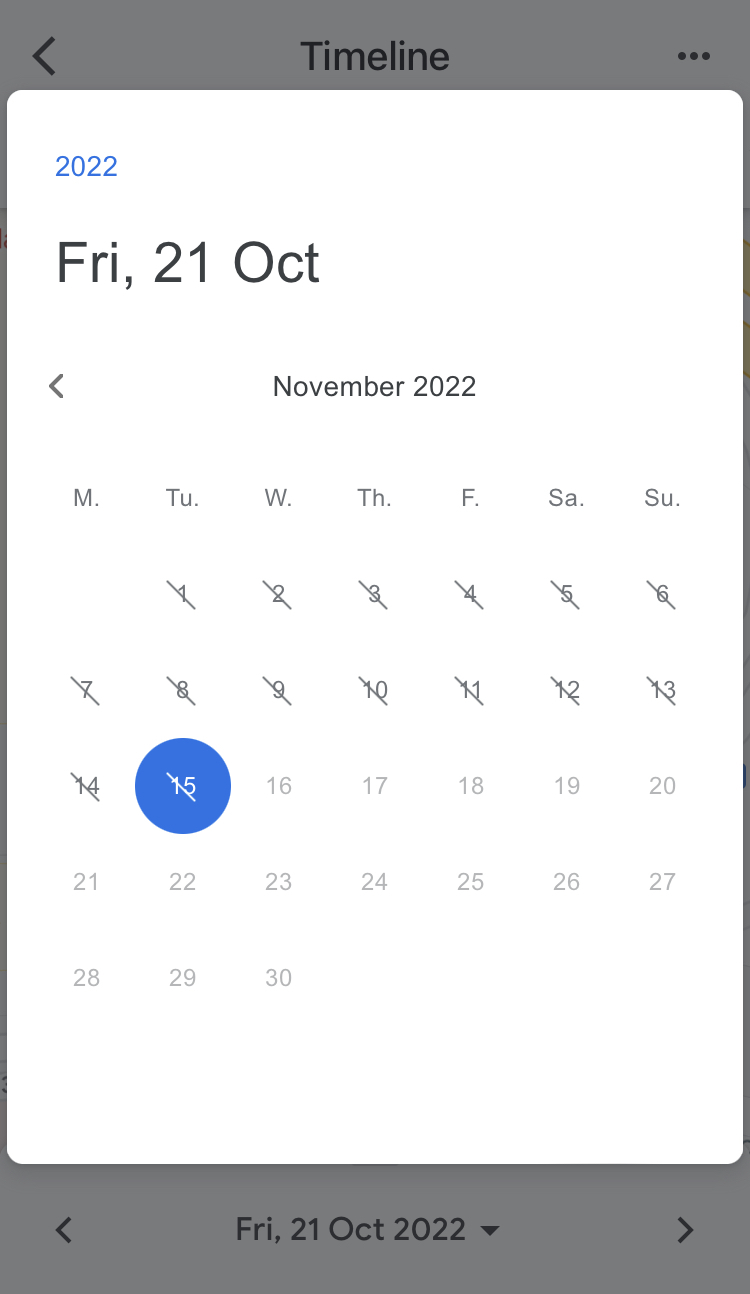This is a detailed screenshot taken on a phone or tablet. It features a substantial white overlay box dominating the center of the screen. In the upper left corner of the overlay is a small print indicating the year, "2022." Below that, in prominent black font, the text reads, "Friday, 21 OCT," which stands for October 21st. Adjacent to this, a small black arrow points to the left. On this same line, "November 2022" is clearly displayed, with the days of the week abbreviated as M (Monday), T (Tuesday), W (Wednesday), T (Thursday), F (Friday), S (Saturday), S (Sunday). The calendar for November shows that the month begins on Tuesday, the 1st.

From the 1st to the 15th of November, each date is crossed out, indicating past days. The dates from the 16th to the 30th are slightly grayed out, signifying upcoming days. A blue circle highlights the 15th, marking it as the current day. In the background, underneath the overlay, the word "Timeline" is visible in black letters at the top of the page. At the bottom, "Friday, 21st October 2022" is repeated, mirroring the date displayed in the overlay box.